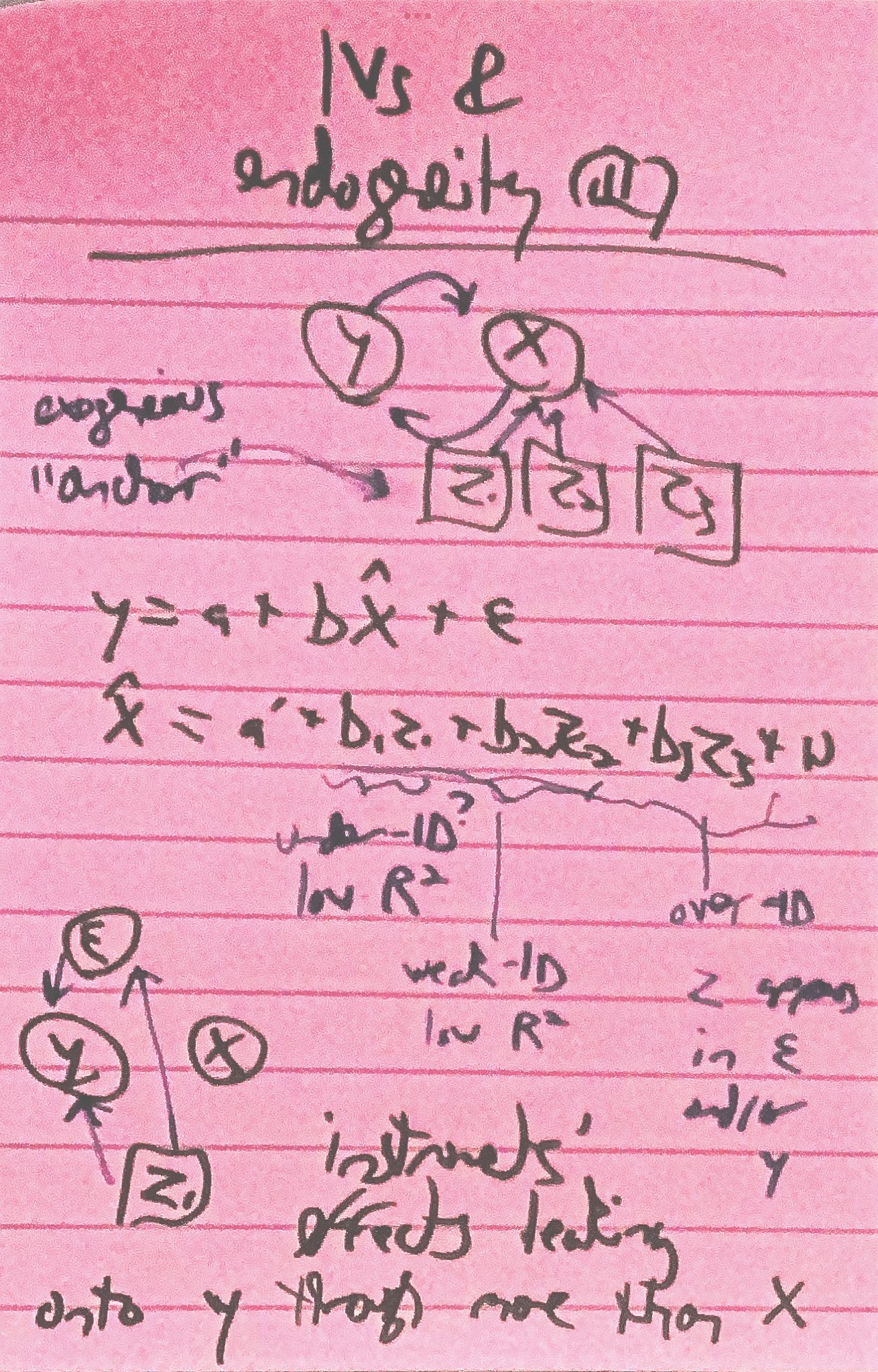This is an image of a pink piece of notebook paper densely filled with black writing. Much of the text is in cursive and difficult to decipher. At the top, the words "IBS" and a partially readable term that seems to start with "endo" and end with "itty" are visible. Below this header, there is a symbol followed by the underlined text "XO" and possibly the word "anchor" with exclamation points.

The paper also contains several mathematical notations. One prominent section includes "Y" within a circle, and an arrow pointing to the letter "X". Additionally, "Z1", "Z2", and "Z3" are enclosed in squares, pointing towards the "X", which in turn points back to the "Y".

Among the equations, there is one that reads "Y = A + B + E" (though the placement of "times" suggests a multiplication operation might be implied). Another equation involves "X", represented with a triangle symbol above it, reading as "X△= A/ + B1Z1 + B2 (possibly Z2) + B3Z3 + ...", with more symbols scattered throughout the page.

Overall, the paper is filled with an array of notations, equations, and symbols, creating an intricate and complex mathematical or theoretical exposition.